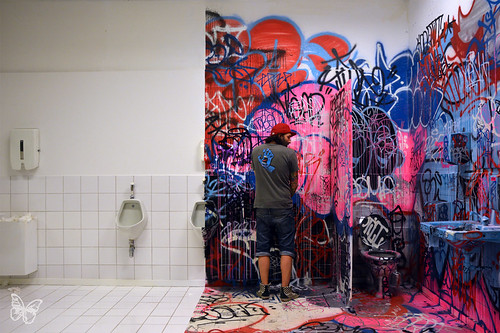The image depicts a surreal bathroom scene split evenly down the middle. The left half of the bathroom features pristine white tiled walls and floor, accompanied by spotless white urinals. A sleek white wall with a butterfly logo can be seen in the bottom left corner. In stark contrast, the right half is a vibrant canvas of graffiti, with an explosion of colors including pinks, blues, reds, and blacks covering every surface. The graffiti extends to the walls, floor, urinals, a toilet in the far-right corner, and a now primarily blue sink. A person stands centrally against the graffiti-covered wall with his back to the camera. He sports a red baseball cap over long black or brown hair, a gray shirt adorned with blue imagery, jeans rolled up to his knees, and sneakers. The contrasts between the stark white cleanliness on the left and the chaotic, colorful graffiti on the right create a striking visual dichotomy.